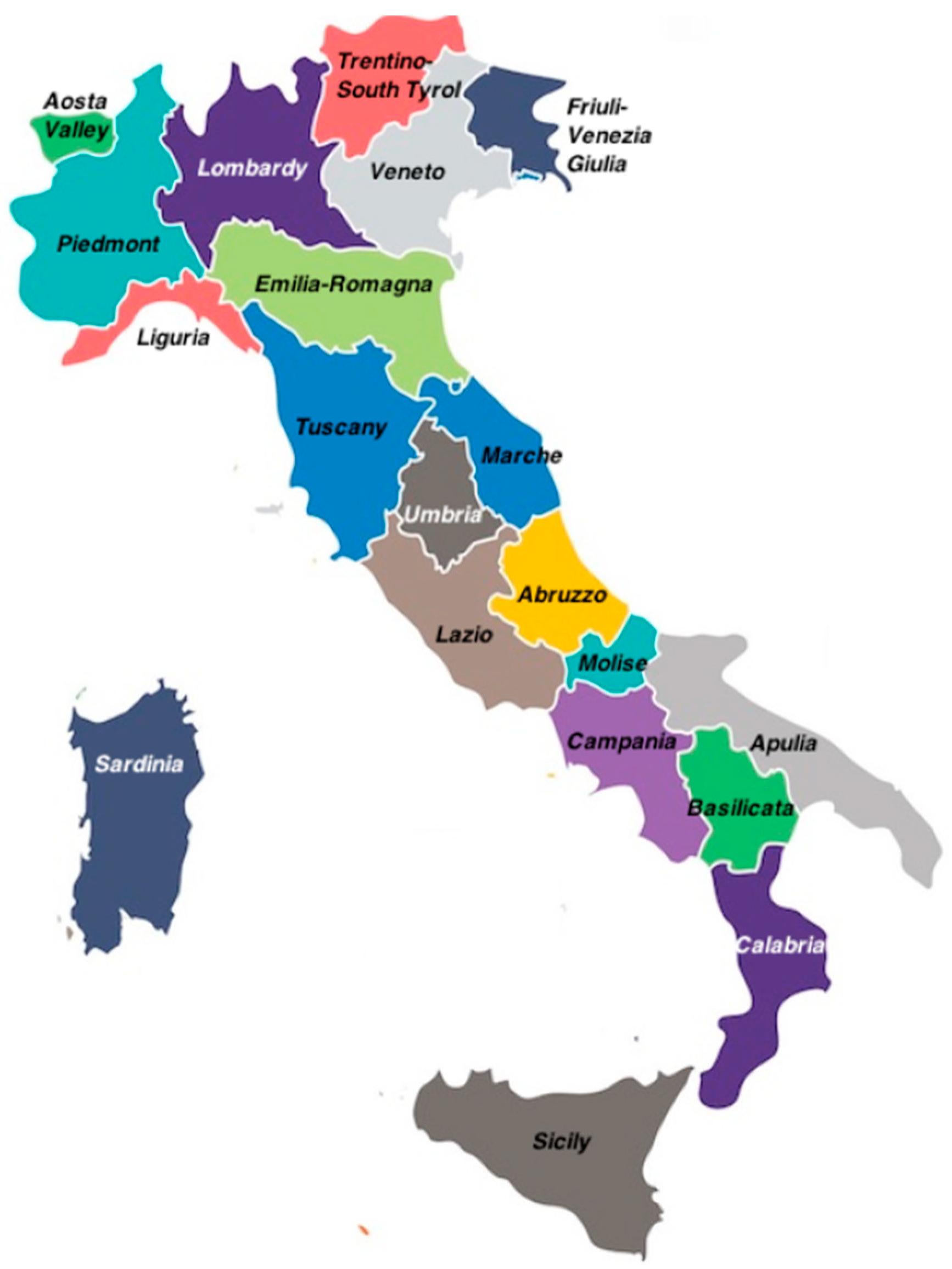This detailed segmented map of Italy highlights the various regions, each distinctly colored to differentiate them. The map features vibrant shades, including greens, blues, pinks, grays, browns, and purples. Prominent regions such as Calabria, Sicily, and Sardinia are clearly marked, along with the Aosta Valley, Piedmont, and Liguria towards the north, extending all the way down to Apulia and Calabria in the south. Sicily sits just below Calabria, and Sardinia is positioned to the far left. The map is designed for educational purposes, perhaps intended for a textbook, and presents Italy without any surrounding ocean, set against a plain white background.